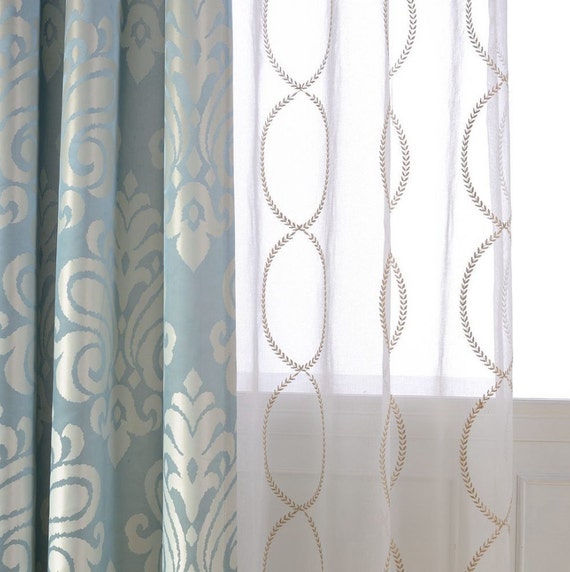The photograph captures a window covered by two distinct styles of curtains. The window, occupying the upper right third of the image, emits an overexposed, bright white light. The lower portion reveals a darker white wall. Draped across the window is a sheer white curtain, intricately embroidered with curving, intersecting vertical lines resembling a linked chain. Next to it, on the left, is a solid, powder blue curtain adorned with silver accents in abstract floral patterns, reminiscent of the French fleur-de-lis. Both curtains appear wavy and creased as if pulled to the side, with the sheer white curtain allowing significantly more light to pass through compared to its opaque counterpart.